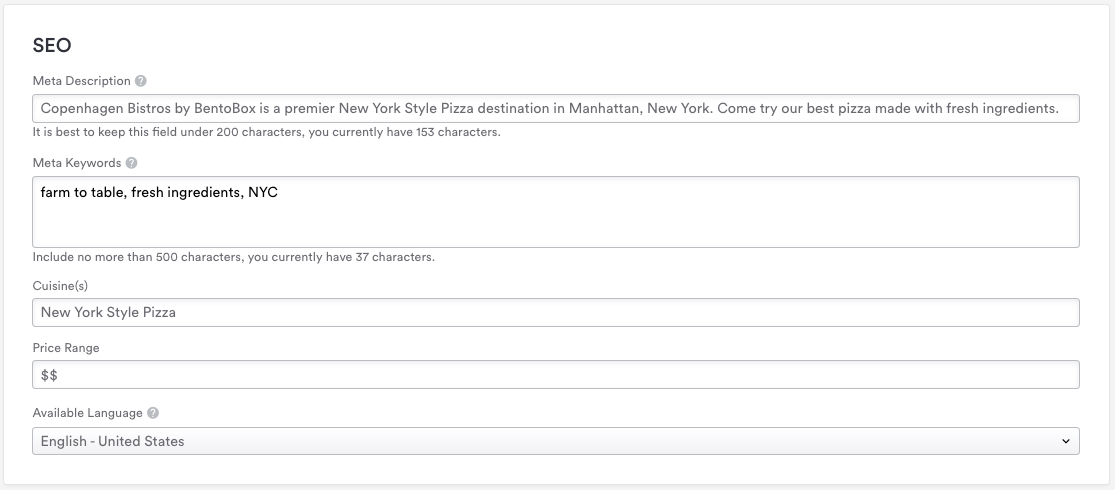Screenshot of SEO settings for Copenhagen Bistros by Bento Box, a premier New York-style pizza destination in Manhattan, New York. The top of the page displays "SEO" in bold, capitalized black letters. Below it, a white text box contains the meta description: “Copenhagen Bistros by Bento Box is a premier New York style pizza destination in Manhattan, New York. Come try our best pizza made with fresh ingredients.” A note below indicates, “It is best to keep this field under 200 characters. You currently have 153 characters.”

Next, the "Meta Keywords" section lists keywords in another white text box: "farm to table fresh ingredients, New York City," with a reminder to include no more than 500 characters, currently using 37 characters.

Further down, the "Cuisine" is specified as "New York style pizza," and the price range is denoted as "$$". The available language is listed as "English, United States."

The text throughout the page is primarily in black and white, with some sections appearing in a grayish tone after typing. This setup is designed to help users optimize their search engine visibility for the restaurant, ensuring key elements are easily searchable for potential customers.